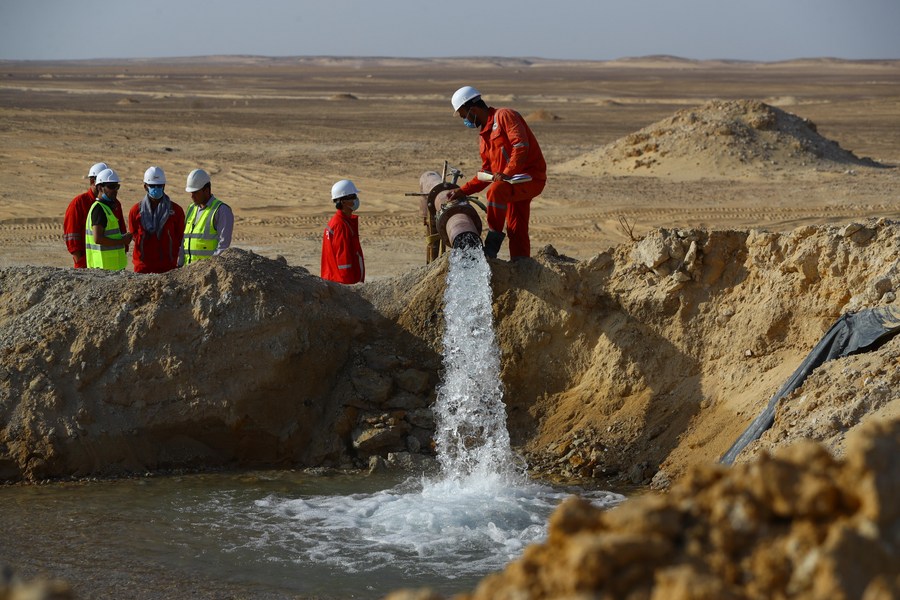In this photograph, six workmen are engaged in an operation in a vast, flat, desert-like field filled with dirt mounds and piles. The landscape is dominated by dirt, with piles scattered across the area and a man-made hole lined with plastic. The majority of the sky is cropped out, leaving a thin strip of overcast grey sky framing the scene. Two workmen are operating a valve to pump water through a large pipe into the hole. All six men wear white construction helmets, and their attire includes red jumpsuits for four of them and yellow-green high-visibility vests for the remaining two. Most of the workers are wearing masks to protect themselves from the dirt, except the two in high-visibility vests who are discussing the situation. The men appear to be conducting a drilling operation perhaps aimed at either filling the pit with water or continuing to excavate until they reach an aquifer. The overall setting implies a methodical and coordinated effort amidst the stark, dirt-filled expanse.